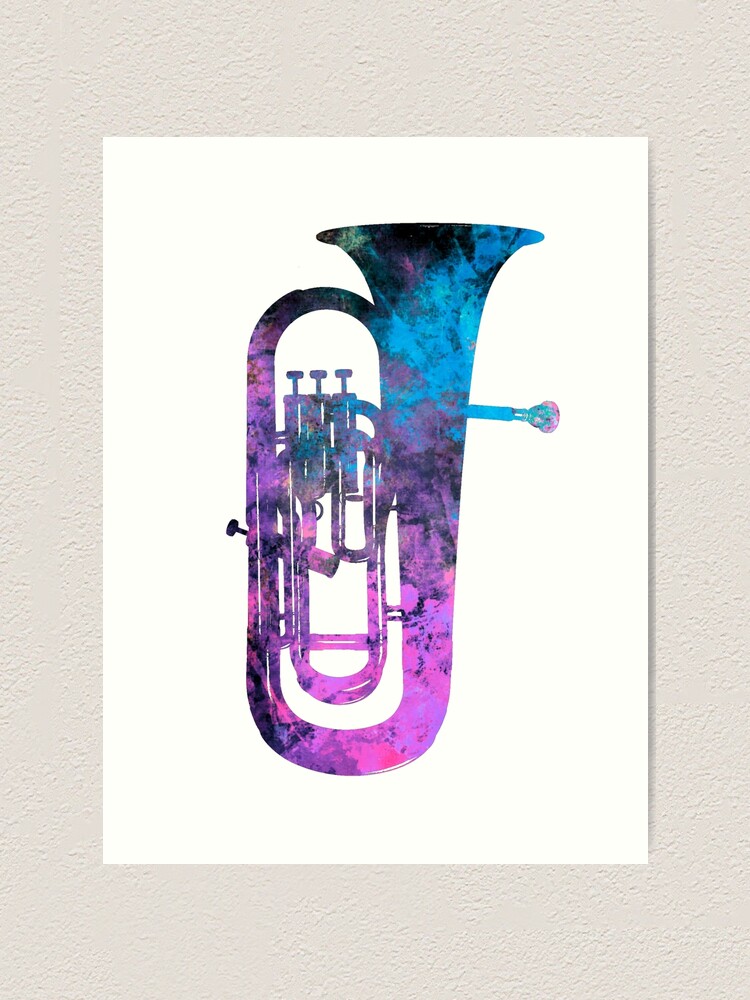The image features a detailed, striking watercolor illustration of a brass instrument, most likely a tuba or a saxophone, positioned upright with its bell facing upwards. The instrument is depicted in a tie-dye array of colors, predominantly rich blues, vibrant pinks, deep purples, stark blacks, and crisp whites. This vivid illustration, characterized by its intricate and controlled watercolor technique, fills the center of a plain white sheet of paper. This single sheet is hung centrally on a piece of textured, eggshell-colored drywall, further emphasizing its vibrant color palette against the neutral, warmer background. The instrument's colorful silhouette stands as the focal point in the composition, capturing attention through its elaborate and non-traditional representation.